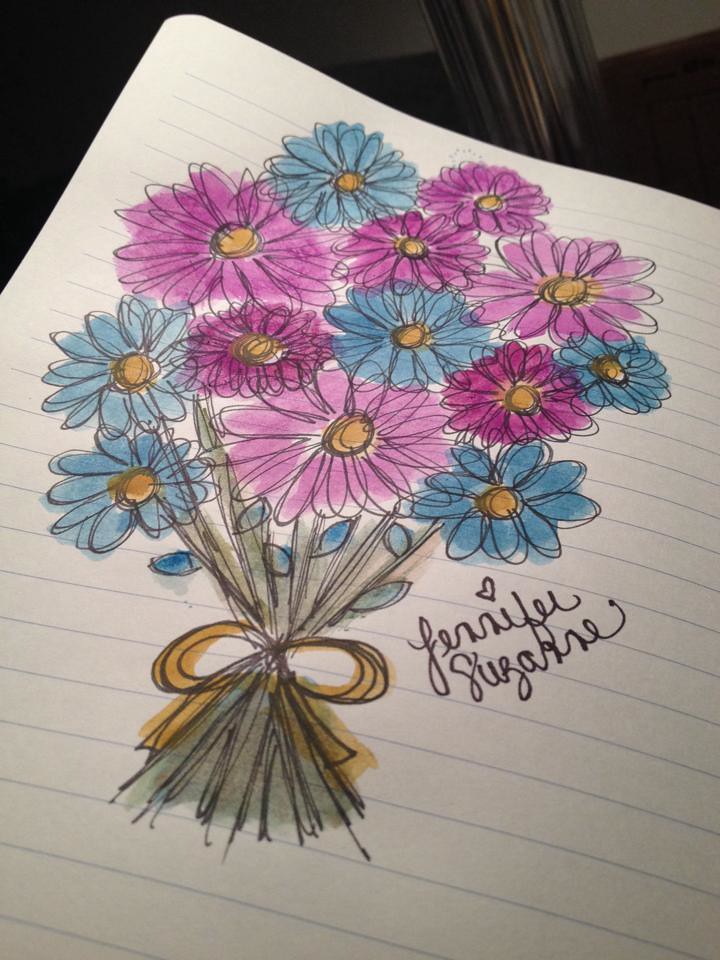This image is a vertically oriented, realistic photograph with a dark background. The top left corner is predominantly black while the top right reveals faint, indistinct shapes. The background features streaks of gray, brown, and black, with a faint white wall and a brown horizontal line at the base. The main focus is a slightly off-white, wide-ruled notebook page with light blue lines, exhibiting slight waves indicating it might still be attached to a notebook.

The notebook paper showcases a hand-drawn bouquet of flowers. The illustration, which appears to be made with a mix of ink, pencil, and colored markers or paint, is not professionally done but charmingly detailed. The bouquet features approximately 20 flowers in pink, purple, and blue, each with black outlines and somewhat mismatched painted colors within. Each flower has a yellow center and is tied together by a yellow bow, with the stems extending through and below the bow.

Towards the bottom right of the page, there is a cursive signature reading "Jennifer Suzanne," with a heart dotting the 'i' in Jennifer. The drawing conveys a heartfelt, handmade quality, making it an endearing illustration despite its lack of precision.